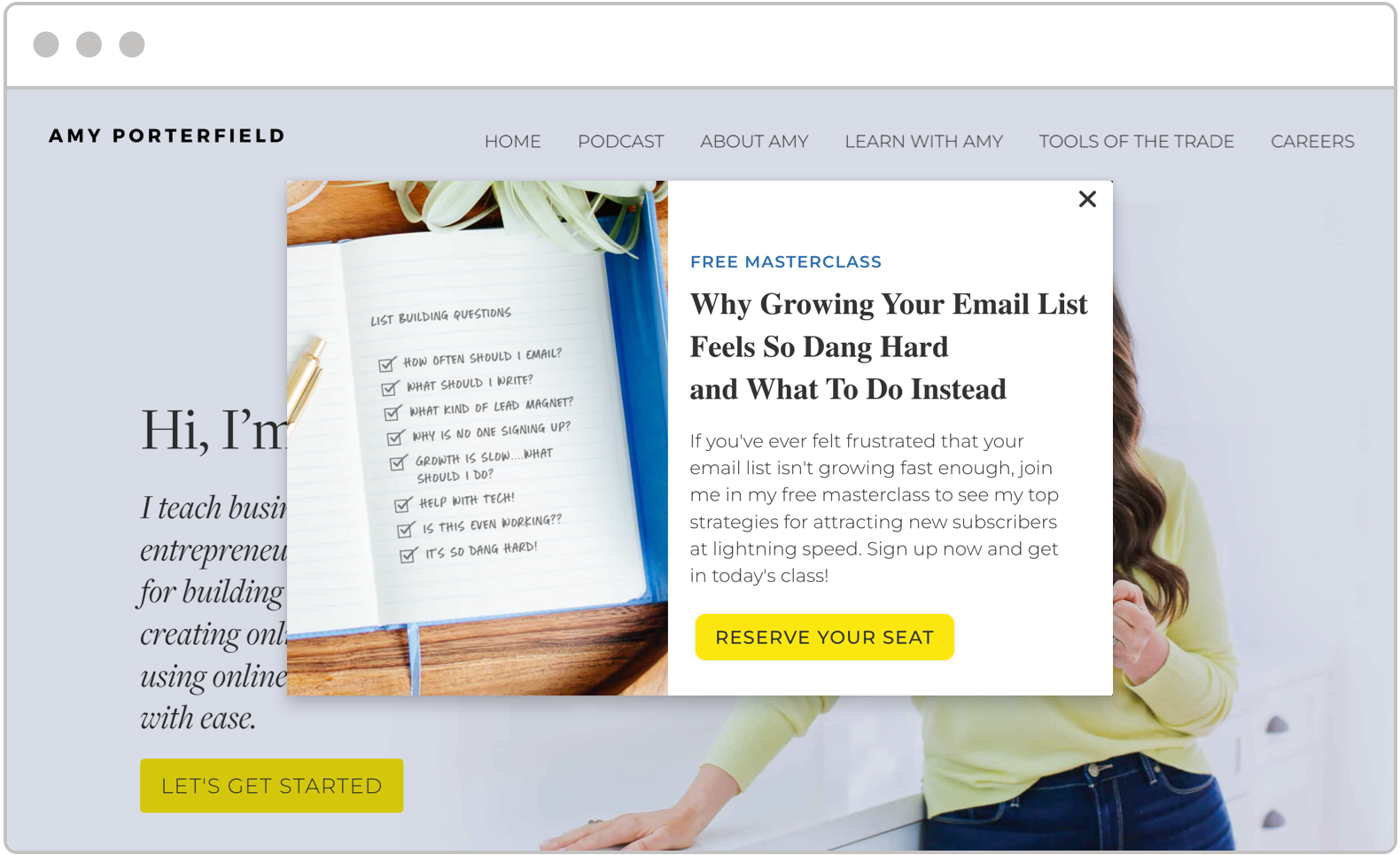The web page dedicated to Amy Porterfield features a clean and organized layout. At the very top, a white border hosts three subtle gray dots. The background of the webpage is entirely gray, with black lettering providing strong contrast for readability. In the top left corner, "Amy Porterfield" is prominently displayed, alongside a horizontal navigation bar offering six categories: Home, Podcast, About Amy, Learn with Amy, Tools of the Trade, and Careers.

Centrally positioned is an engaging pop-up box. On the left side of this box, an image resembling a notebook or diary introduces a section titled "List Building Questions." Each question listed here is accompanied by a checkbox, all visibly marked with check marks. On the right side of the pop-up, an invitation to join a free masterclass is highlighted. It reads: "Free Masterclass: Why Growing Your Email List Feels So Dang Hard and What to Do Instead. If you've ever felt frustrated that your email list isn't growing fast enough, join me in my free masterclass to see my top strategies for attracting new subscribers at lightning speed. Sign up now and get in today's class." A vibrant yellow rectangle at the bottom of the pop-up carries the call-to-action text "Reserve Your Seat" in bold black letters. The pop-up can be closed by clicking a black 'X' in the top right corner.

In the main background, an image provides a subtle yet effective visual element. The picture depicts a woman, presumably Amy Porterfield, standing against a kitchen counter. Although her face is not visible, her long brown hair, yellowish long-sleeve top, and blue jeans are evident. Accompanying the image, partial text reads: "Hi, I'm," followed by incomplete phrases such as "I teach business," "entrepreneur," and "for building creating online using online with ease." Directly below the text, another yellow rectangle appears with the phrase "Let's Get Started" in black lettering.

This thoughtfully crafted layout and the detailed pop-up box create an inviting experience for visitors interested in learning more about Amy Porterfield's business strategies.